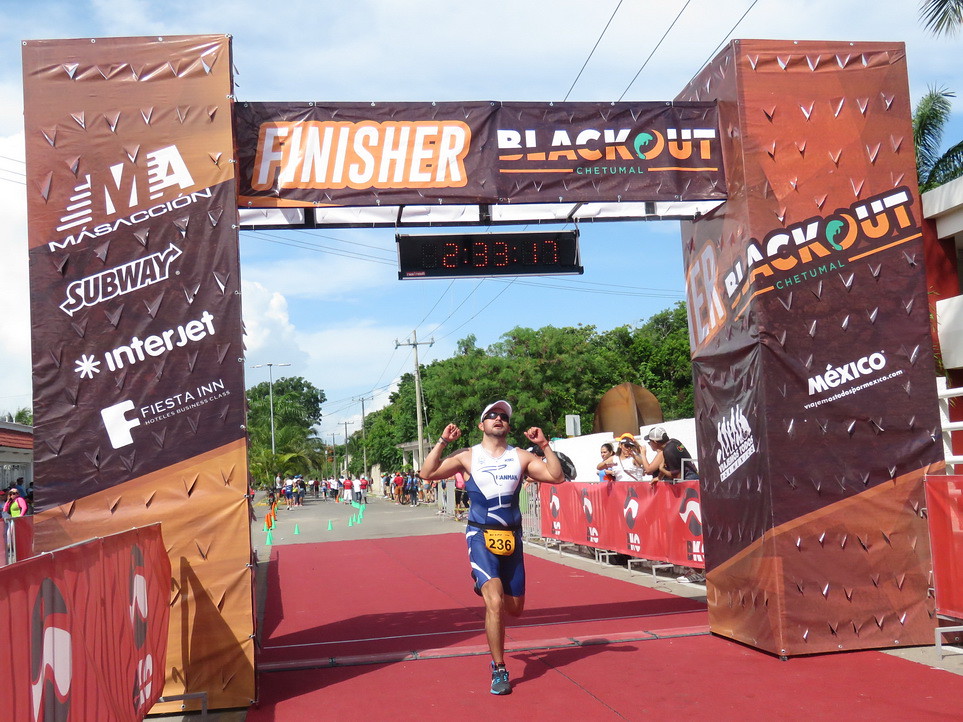In this vivid photograph capturing the finish of a footrace in Mexico, a male runner, wearing blue shorts and a matching blue top with a white bib, triumphantly crosses the finish line, marked by towering rectangular structures approximately 15 feet tall. The banner overhead reads "FINISHER" on a yellow background and "BLACKOUT" on a purple background, with "CHETUMAL" in blue letters. His race bib proudly displays the number 236. The setting is an open street race, with the pathway lined by fences adorned with advertisements for brands like Subway, Interjet, and Fiesta Inn. A digital chronometer beside the finish line indicates the runner's time as 2 hours and 33 minutes, a commendable marathon completion time. The road is decorated with various colored cones—green, red, light brown, and dark brown—and flanked by green trees and wooden telephone poles under a clear blue sky. Spectators can be seen cheering from the sides, adding to the celebratory atmosphere as the elated runner raises his hands to his shoulders in a victorious gesture, savoring his accomplishment.